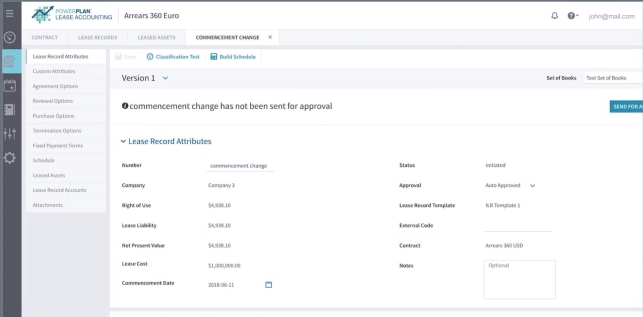A screenshot from a web page titled "Power Plan Lease Accounting" features a left sidebar with multiple icons aligned vertically. The main content area highlights a section titled "Version 1" in black text, followed by a note stating "Commencement Change has not been sent for approval." Beneath this, in blue text, the section titled "Lease Record Attributes" lists several fields: Member, Company, Right of Use, Lease Liability, Net Present Value, Lease Contract, and Commencement Date, with an example date of 2018-06-11. On the right side, there is a teal-colored button labeled "Send for A," though the text is partially cut off.